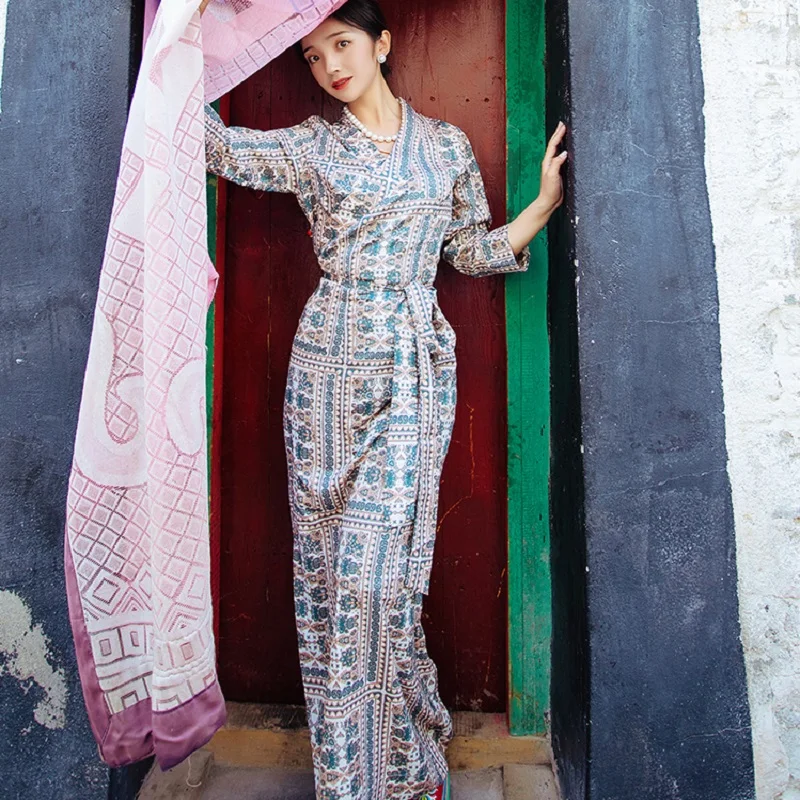In this striking photograph, a young Asian woman is elegantly posed in a doorway, holding back a richly designed curtain with her right hand. The curtain, adorned with a diamond pattern and purple trim, adds a touch of vibrancy with its pink hues. She is dressed in a distinctive white and blue dress featuring a cross stripe pattern, with a vertical blue stripe down the center interspersed with horizontal stripes approximately every foot, creating a visually captivating ensemble. Her left hand, with fingernails painted white, rests against a black wall made of stone or brick, which has a noticeable white smear of paint on the left side. She accessorizes with a classic white pearl necklace and matching earring, and wears bright red lipstick that adds a pop of color to her serene, poised demeanor. Her dark hair, styled in a ponytail or bun, complements her youthful appearance, marked by her early 20s. Behind her, the doorway is framed by a green trim, leading to a brown wooden door that contrasts beautifully with the dark, somber tones of the walls around her.